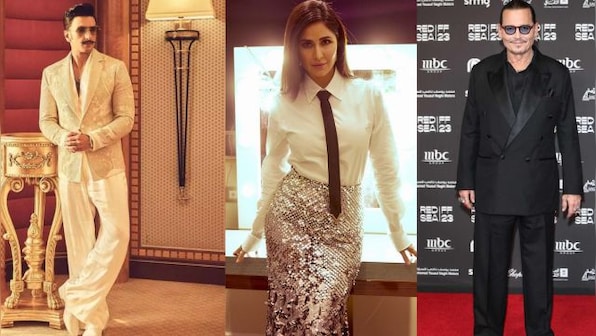This composite photograph features three distinct sections, each showcasing a notable figure. On the far right, Johnny Depp is seen on the red carpet for the Red FFC 23 event, donning a black tuxedo, black pants, and sunglasses with his hair slicked back. The backdrop features the NBC logo among other sponsors. In the center, a woman sporting a white button-up shirt and a sequined skirt, tied with a long dark tie, gazes directly at the camera with a partial smile. She is seated on a countertop, leaning back towards an illuminated backlit mirror reminiscent of a dressing room. To the left, another male figure stands in an ornate room. He wears loose, billowing white pants, a cream-colored blazer over a red shirt, and sports a handlebar mustache with a pompadour hairstyle and sunglasses. Leaning against a gold-painted wooden table, he stands in front of an opulent light fixture with a black stem and an orange frame.